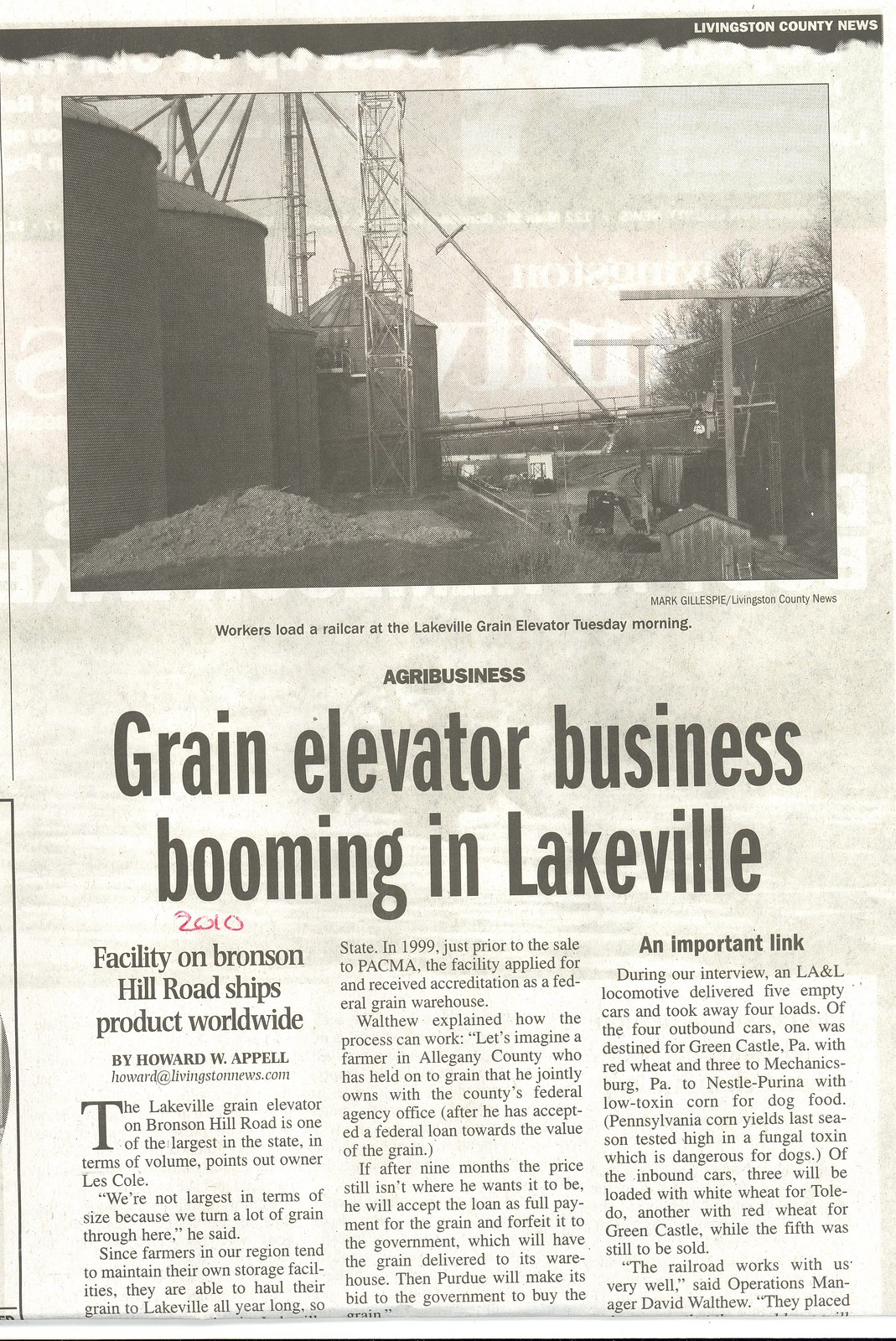This black-and-white image captures a newspaper article from the Livingston County News, headlined "Green Elevator Business Booming in Lakeville." The article, authored by Howard W. Appel, details the operations of the Lakeville Grain Elevator located on Bronson Hill Road, noted for its high volume of grain despite not being the largest in size. The facility, which ships products worldwide, received federal grain warehouse accreditation in 1999, just before being sold to PACMA. The accompanying photograph by Mark Glipsy shows workers loading a rail car at the Lakeville Grain Elevator, illustrating the bustling activity described in the piece. During the interview, an LA&L locomotive delivered five empty cars and took away four loads, with destinations including Greencastle and Mechanicsburg, Pennsylvania.